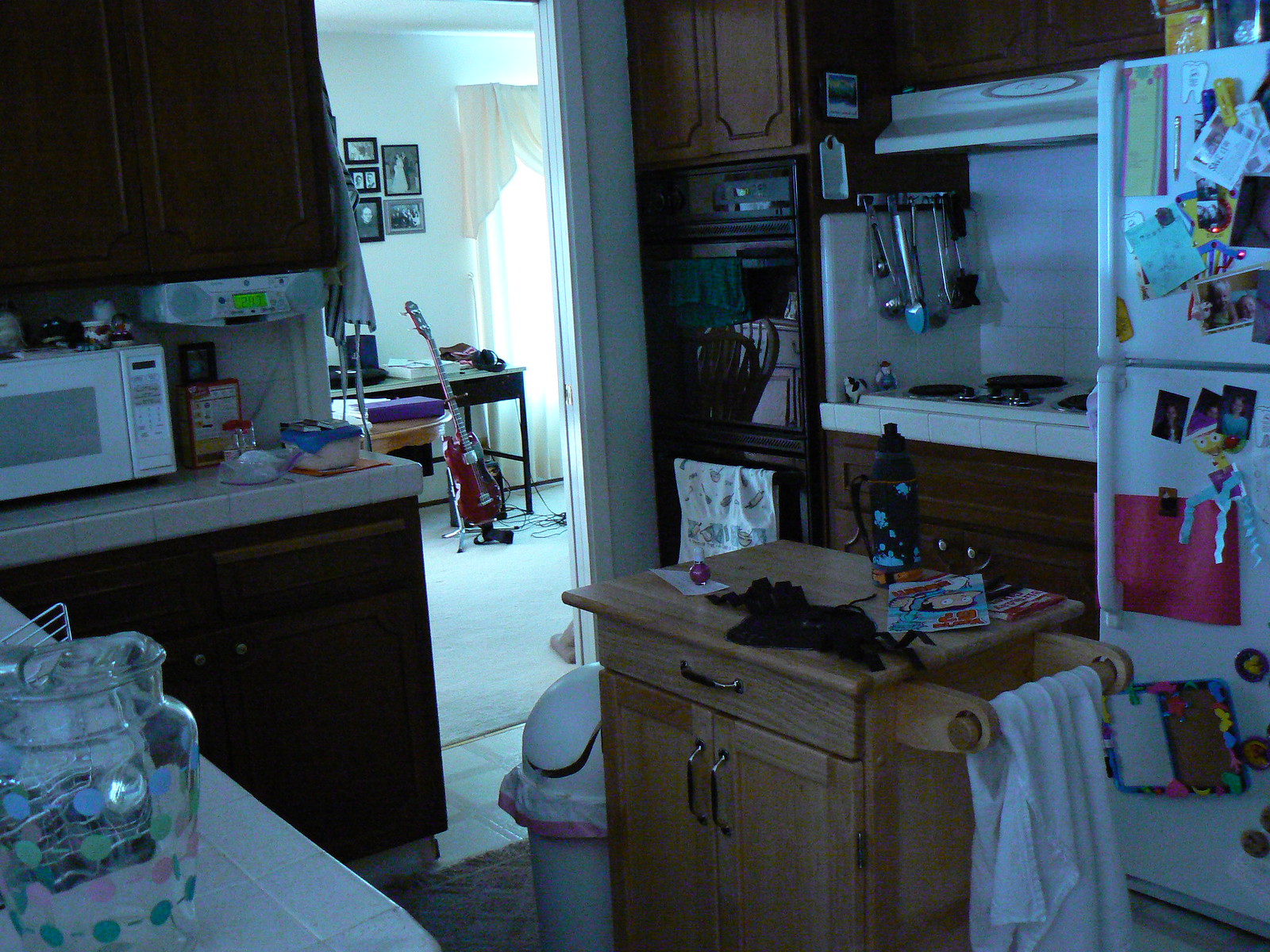In this photograph, we are presented with a detailed view of the interior of a walk-in kitchen area. Dominating the center of the kitchen is a wooden counter, serving as a small vanity or island. Attached to this counter on the right side is a dowel from which a white towel is hanging. Atop this wooden counter lies a magazine or comic book in the top right corner and a water bottle positioned centrally.

Adjacent to the left of the wooden island is a white plastic trash can, complete with a plastic trash bag inside. In the bottom left-hand corner of the image sits a jar, possibly containing coins. Moving to the top left part of the photograph, a white microwave is perched on a kitchen counter, with a Tupperware container storing food placed just to its right.

The far right side of the image showcases a tall white refrigerator, its doors festooned with various pieces of paper, magnets, and photographs. Positioned to the left of this refrigerator is a stovetop and grill area, with a metal rack hanging utensils on the adjacent wall. Above this cooking area, we see air vents providing ventilation. Further to the left sits an elevated oven that stands prominently above the ground.

Extending beyond the immediate kitchen area into another room, the image captures a scene with white carpeted flooring and an electric guitar standing against a wall. This additional space features several other items including a desk, contributing to the comprehensive domestic setting.